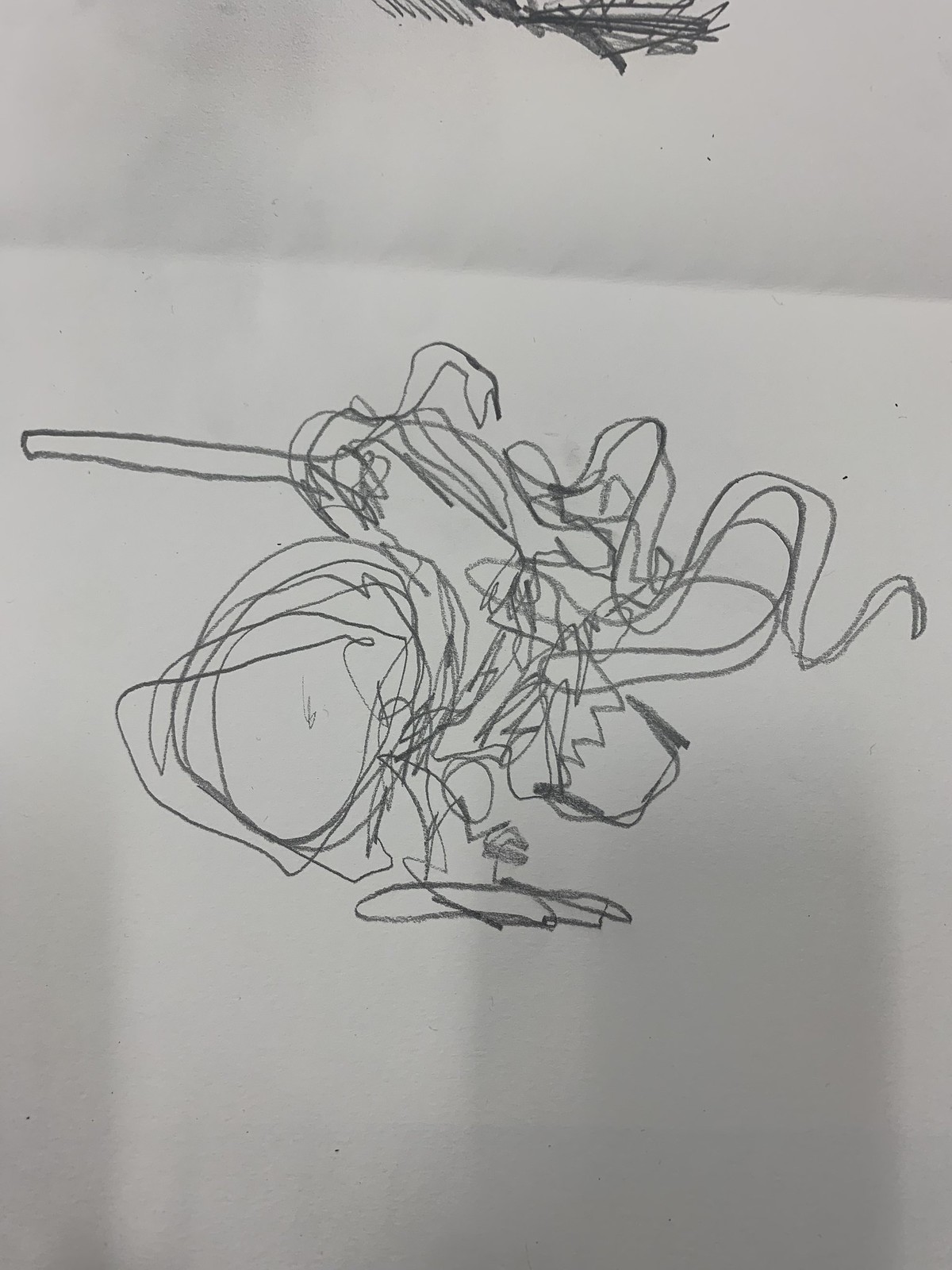The image features a white sheet of paper that dominates the entire frame. At the center of the paper, there is a dense and intricate mass of pencil scribbles. These central scribbles appear concentrated, with a circular area on the left side and a bar-like extension that reaches outward to the left. Additionally, the center contains a cluster of jagged lines, giving it a chaotic texture. Towards the top of the image, there is another patch of scribbles that are more condensed and only occupy the middle section, partially cropped off by the top edge of the paper. The section on the left side of the central mass has more spread out and thinner lines, while the right side features wavy patterns mingling with the jagged center. The overall effect is a complex and dynamic composition of pencil lines.